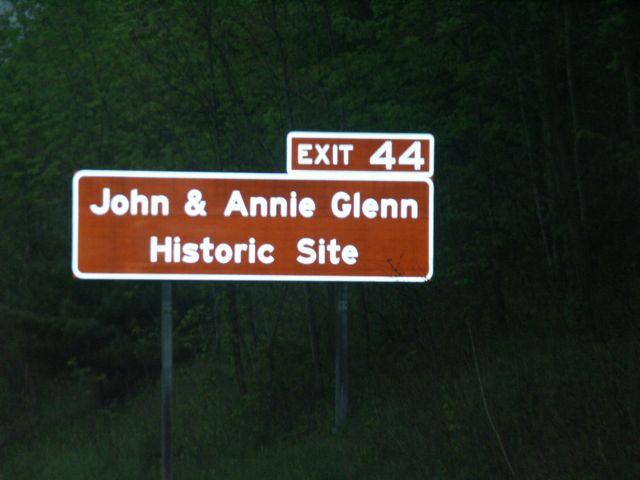This photograph, likely taken at night or dusk due to its overall darkness, features a prominent roadside sign indicating the "Exit 44, John and Annie Glenn Historic Site." The image captures a rural, heavily wooded area dominated by various trees, including deciduous types and at least one pine. The dark brown sign, with white bold text, is mounted on wooden poles set into the ground and has a smaller, matching brown rectangle indicating the exit number. There seems to be a slight and faint visible sliver of sky peeking through the top left corner of the frame. The steel legs of the sign appear somewhat rusted and blackened, hinting at age or wear. Below the sign, patches of grass are visible, adding to the natural setting of the scene.